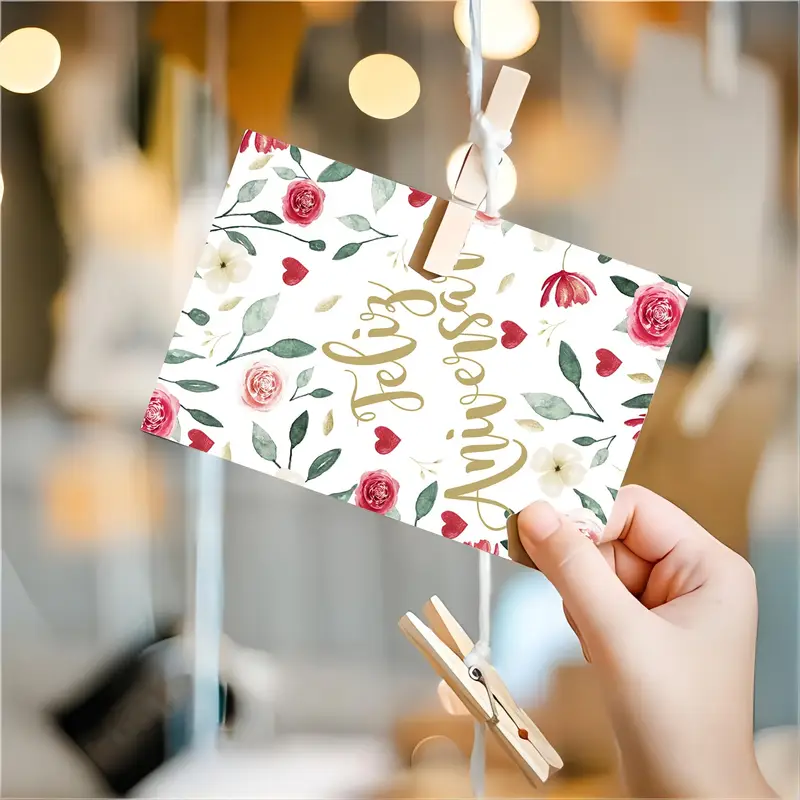The image depicts a white greeting card adorned with pink flowers and green leaves, held between an individual's thumb and second and third fingers on the right-hand side of the frame. The card, which features the gold text "Feliz Anniversary," is also suspended by a brown wooden clothespin attached to a white string, hanging vertically from above. The background is blurry, revealing faint details such as lights, and what appears to be a white couch with a black pillow in the left-hand corner. The overall ambiance of the room is blurred with hints of yellow, blue, and white tones. Additional details of the room remain indistinct due to the soft focus.